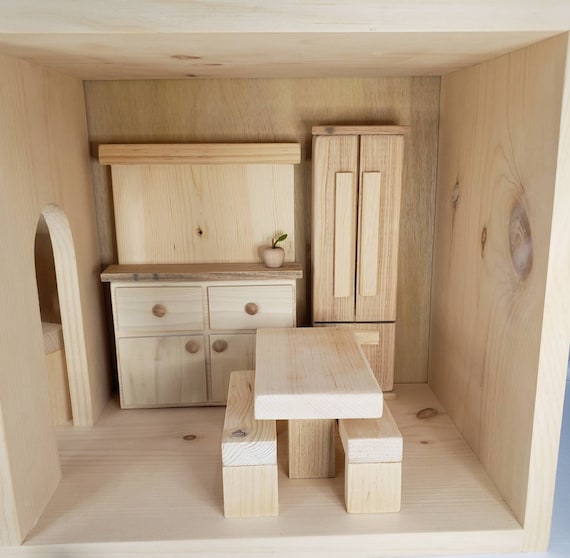This is a vertical rectangular photograph showcasing the interior of what appears to be a model room within a dollhouse, designed to resemble a kitchen. The entire room, including the floor, walls, and ceiling, is crafted from light-colored, unfinished wood, giving it a cohesive, unpolished appearance. Dominating the space is a wooden picnic-style table with sturdy benches on either side, all made from the same light wood. In the front, thick wooden pieces support the benches and table. 

At the back of the room, there's a vertical cabinet featuring a slightly darker wood with a decorative design on its front, and a wider cabinet is positioned to its left. To the right side of the room, there's what looks like a multi-purpose storage piece, potentially a double-doored fridge or wardrobe, also made from wood. This piece includes side-by-side upper doors and a lower section that could represent a freezer.

An arched doorway is visible on the right wall, adding architectural interest to the space. On the countertop, there are small details such as a wooden napkin and a wooden apple with a green leaf. This detailed miniature setup captures the essence of a simple, rustic kitchen, entirely fashioned from light plywood.